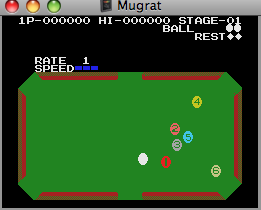This image is a detailed screenshot from a billiards-themed video game. Dominating the upper section of the screen is a gray banner that prominently reads "Mugrat" in the center. To the left of the banner are three circles in red, yellow, and green, resembling traffic light indicators. Just below this banner, the black background features white text displaying "1P-" followed by six zeros, "HI-" also followed by six zeros, and "Stage-01." Additional text reads "Ball" next to two circles, and "Rest" next to two diamonds. Above the billiards table, the text "Rate-1 Speed" appears, with three blue rectangles indicating the speed level. The green billiard table, bordered by reddish-brown bumpers, is depicted with a set of balls in various colors and numbers: yellow, red, blue, pink, gray, and an unnumbered white cue ball. The detailed and colorful layout underscores the game's structured, yet lively simulation of a pool table game.